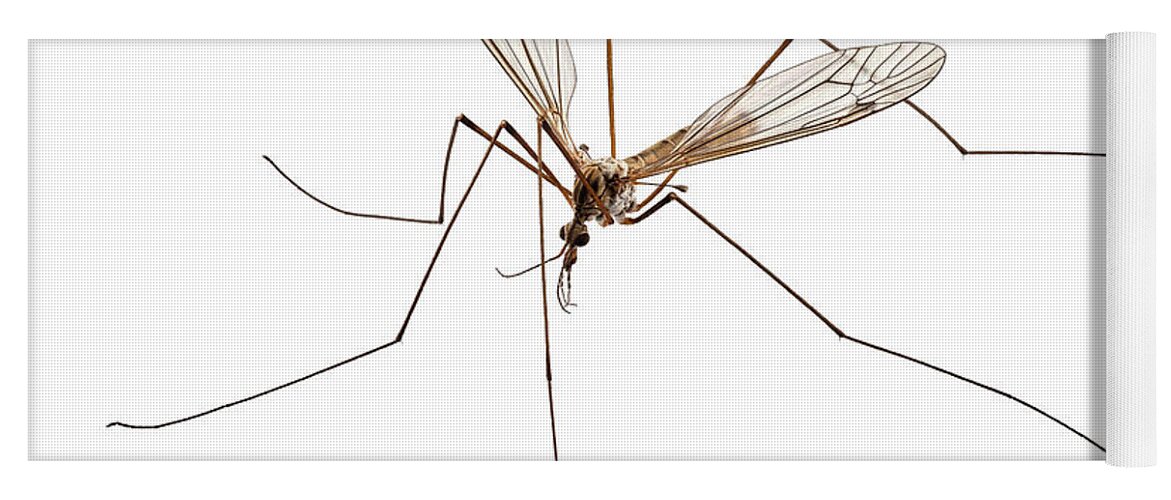The image depicts a detailed, close-up view of a mosquito illustration on a white fabric, possibly mesh or cloth, unrolled horizontally from left to right, resembling a scroll. The white fabric shows subtle mesh texture and the rolling part of it is visible on the right. The mosquito itself is prominently centered, with an elongated brownish body and distinct, transparent wings that are spread out, revealing its legs and body underneath. The head of the mosquito hangs slightly away from its body, connected by a visible neck, and features large, round black eyes with noticeable feelers. The insect has six long, skinny legs, three on each side, and the detailed body includes a segmented shell with tan, brown, and black lines. The intricate design of the mosquito spans much of the fabric, and additional parts of its legs would be revealed if the fabric were further unrolled.